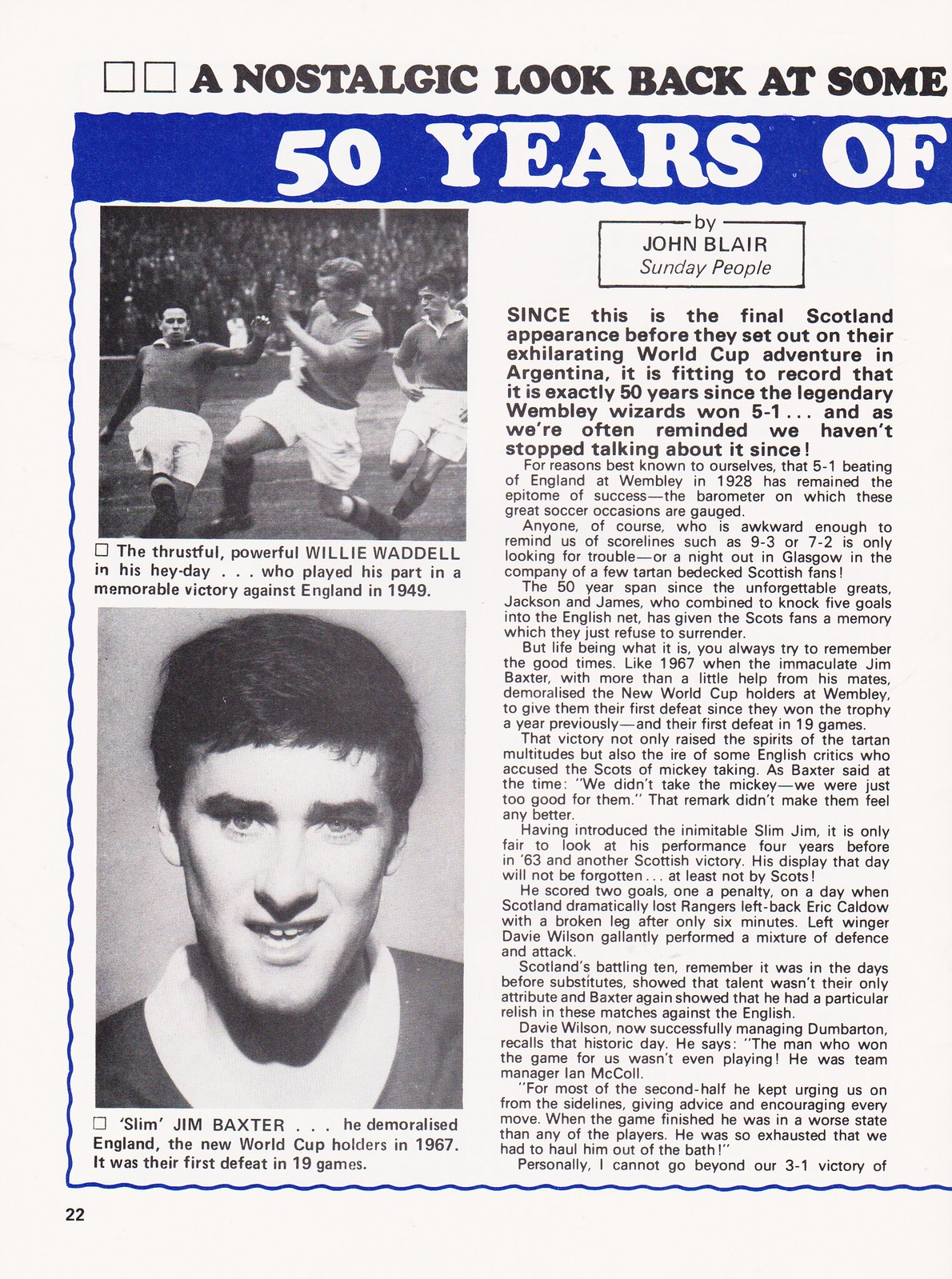This image appears to be an old-time magazine article commemorating 50 years of World Cup soccer. The layout features a nostalgic look back at pivotal moments in soccer history, accented by a black, white, and medium blue color scheme. At the top, the headline in black print states, "A Nostalgic Look Back at Some," though the rest of the sentence is cut off. Directly beneath, a blue banner with white text reads, "50 YEARS OF," continuing the cut-off theme.

To the left, two black and white photographs set the scene. The top photo captures an action shot of three men playing soccer, accompanied by a caption describing Willie Waddle's powerful play during a memorable victory against England in 1949. Below this, a portrait of Jim Baxter, referred to as "Slim Jim Baxter," highlights his impressive performance against England in 1967, leading to their first defeat in 19 games.

To the right of the photographs, a column of text discusses the World Cup and other soccer-related events, set in black text against a white background. The article, written by John Blair of Sunday People, spans about 10 to 12 short paragraphs. It reflects on Scotland's final appearance before their exhilarating World Cup adventure in Argentina, marking exactly 50 years since the legendary Wembley Wizards' 5-1 victory—a feat that continues to be celebrated and remembered. This rich historical recount ties together personal player anecdotes and significant games, emphasizing the deep-rooted passion for soccer through the decades.